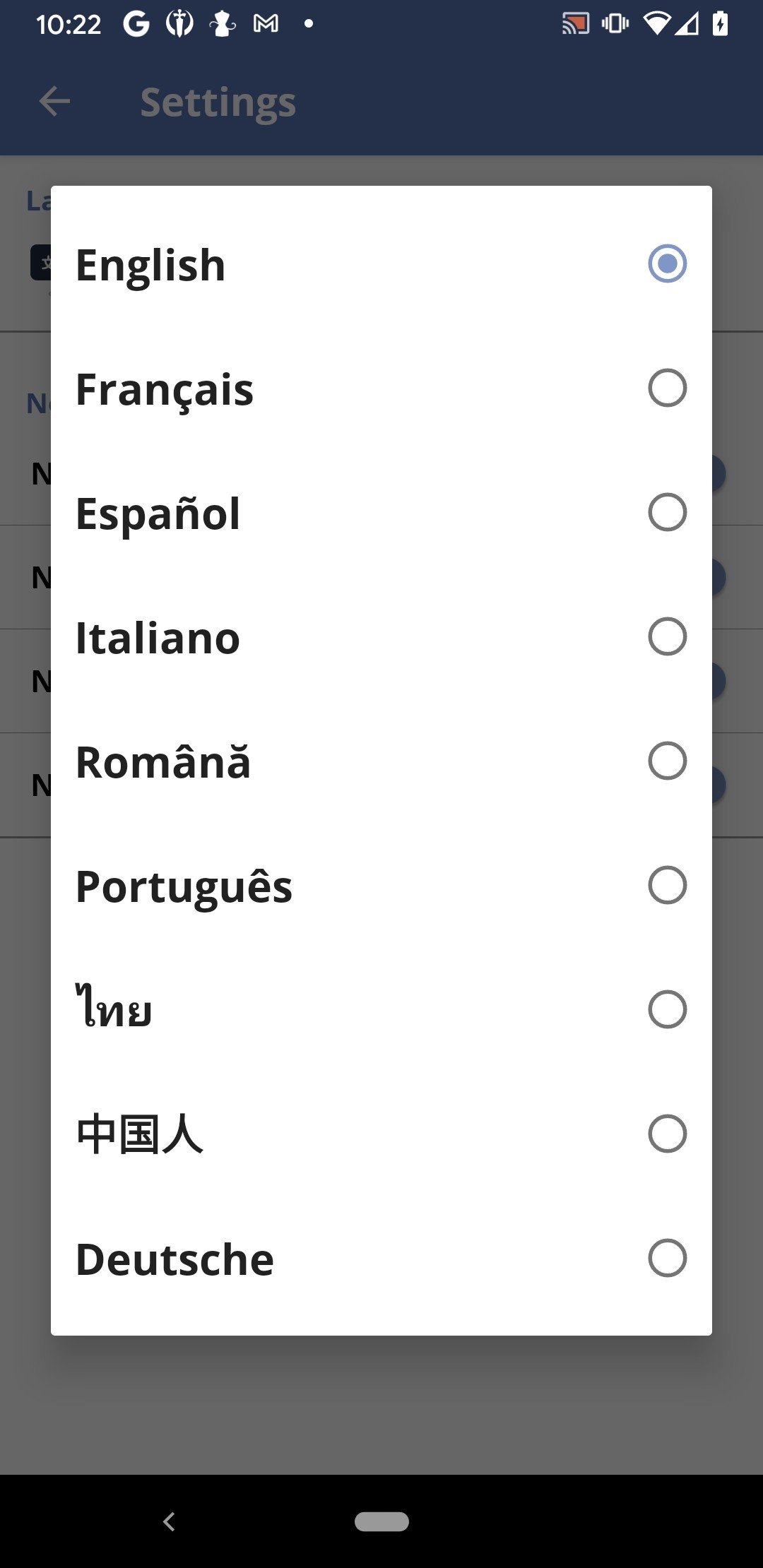A screenshot from a mobile phone displays a prominent pop-up window at the center, occupying most of the screen's height. This pop-up menu features a white background with black text and lists various languages such as English, Français, Español, Italiano, Română, Português, and others, including a language that appears to be "Lelou," some Chinese characters, and "Dush." Small round tick boxes are placed to the left of each language option, and the tick box next to English at the top is marked in blue. 

In the background, partially greyed out due to the focus on the pop-up window, several mobile interface elements are visible at the top. These include the time "10:22" on the left, the Google icon, a red square icon on the right, and indicators for Wi-Fi, mobile signal strength, and battery status. Below this, a settings bar, usually white with a back arrow, is greyed out and positioned underneath the top icons, followed by another whitened-but-greyed panel obscured by the pop-up.

At the bottom of the screen, a thin grey space and a black bar are present, with a small back arrow located about a quarter of the way across the black bar from the left-hand side. Additionally, a small grey rectangle with rounded edges appears in the middle of the bottom bar.